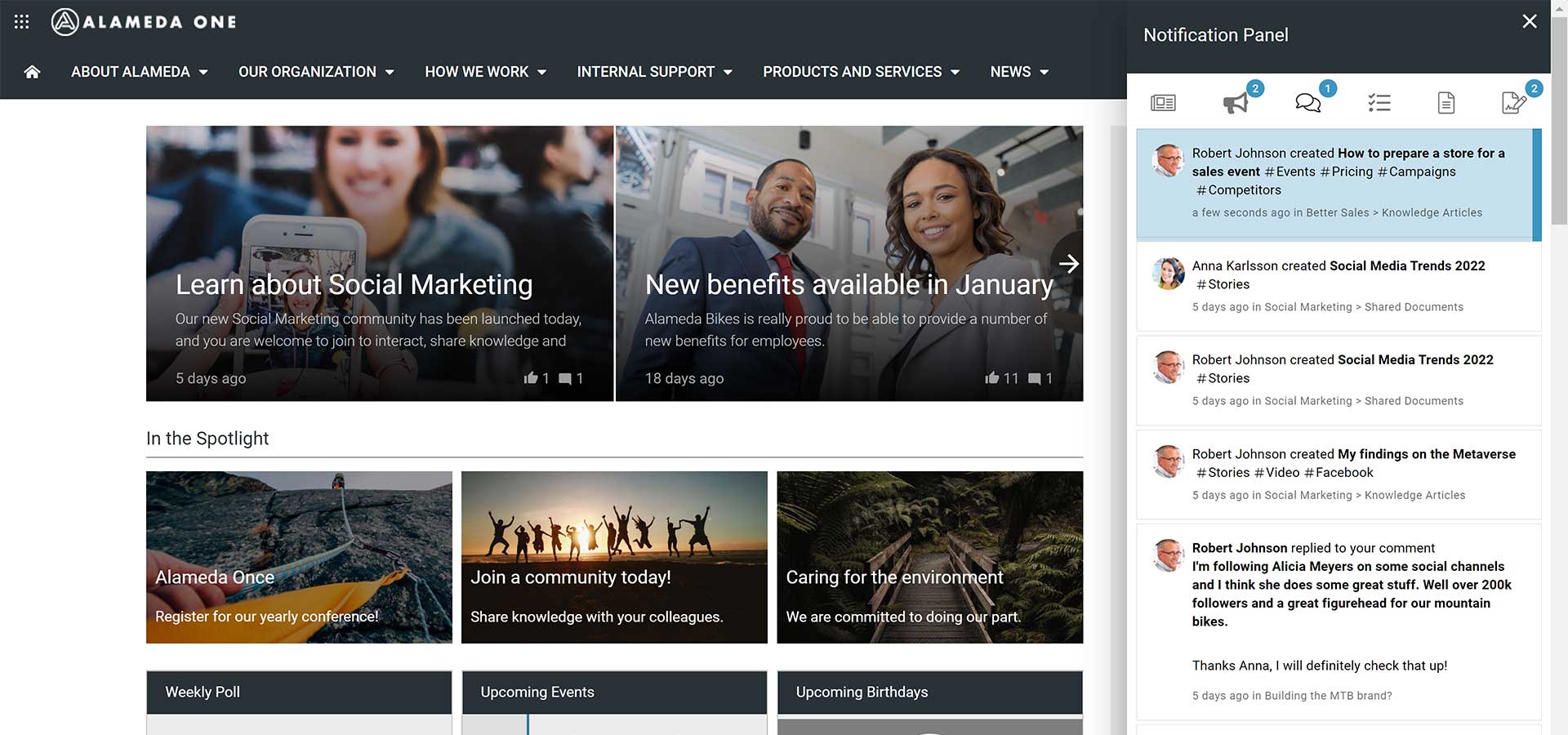The image appears to be a detailed screenshot of a webpage, possibly the internal interface of the organization Almeda. The interface features a black navigation bar at the top with white text listing various sections including "About Almeda," "Our Organization," "How We Work," "Internal Support," "Products We Service," and "News." To the right, there is a notification panel displaying multiple updates:

- Robert Johnson created a guide on preparing a store for a sales event.
- Alan Carlson and Robert Johnson both contributed to discussions on social media trends in 2022.
- Robert Johnson shared stories about his findings in the Metaverse five days ago and replied to a comment.

Additionally, the user mentions following Alicia Meyer, a prominent figure with over 200k followers who is influential in promoting their mountain bikes.

In the center of the page are various images with accompanying text:
- An image shows a phone capturing a woman in the background with the caption "Learn about social marketing."
- Another image of a man and woman with the caption "New benefits available in January."
- An invitation to "Register for a yearly conference" near a mountain climbing scene.
- A promotional image encouraging users to "Join the community today, share knowledge with your colleagues," featuring a group of people jumping against a sunset.
- A commitment to environmental care depicted by an image of a scenic bridge surrounded by trees.

At the bottom of the page are sections for a weekly poll, upcoming events, and upcoming birthdays.